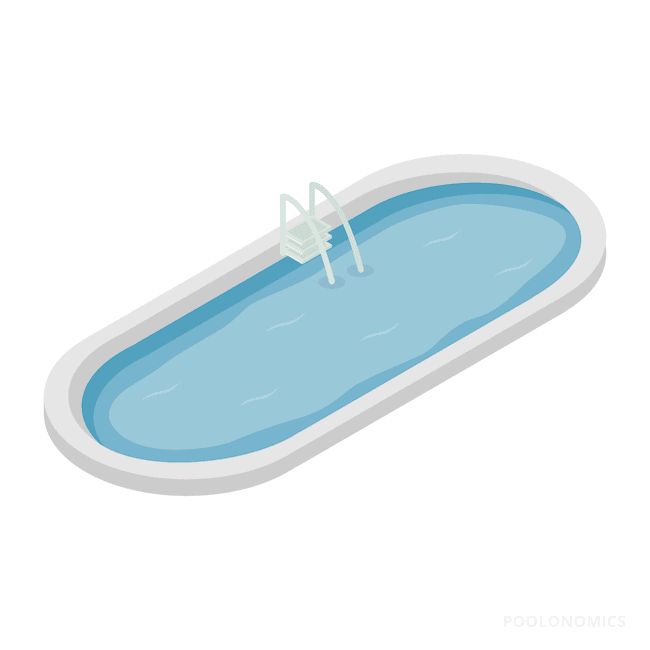This digital illustration depicts an oval-shaped swimming pool, angled from the top right to the bottom left. The pool features a thoughtfully structured gradient of blue shades: the outermost border is the darkest blue, followed by a medium blue middle ring, and the lightest blue water in the center. The surface of the water is adorned with six small white wave lines to indicate movement. Centrally located near the top of the pool is a curved ladder with two rounded handrails and three steps, providing access into and out of the pool. The illustration lacks surrounding context, focusing solely on the pool itself without displaying its environment or background. The art style suggests a cartoonish or game-like quality, similar to what one might find in a Sims game.